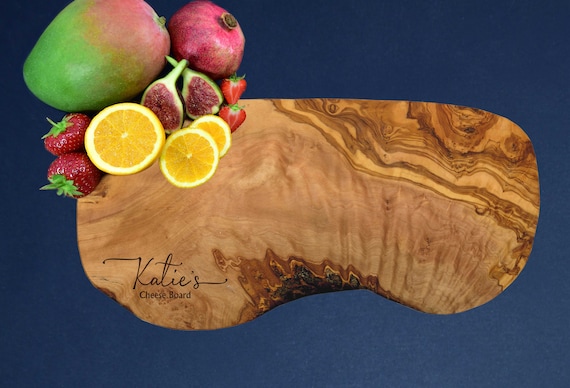This detailed photograph showcases a unique, kidney-shaped wooden cheese board against a dark blue background, which lightens slightly in the bottom right corner. The cheese board is predominantly brown but features striking dark brown and yellow streaks on the top right, highlighting the natural variations of the wood. The board is engraved with "Katie's Cheese Board" in cursive black text at the bottom.

Adorning the cheese board are an assortment of colorful fruits, enhancing its visual appeal. On the left side sits two whole strawberries, followed by three lemon slices oriented upwardly. Behind the lemon slices are two additional fruits, seamlessly transitioning to another pair of strawberries on the right. Dominating the top section, there’s a half green, half red apple, next to a pink fruit, and further complemented by fruit images including a mango, pomegranates, and slices of orange. This layout suggests a marketing display, possibly for an online listing, emphasizing the cheese board's customizable potential and elegant design.